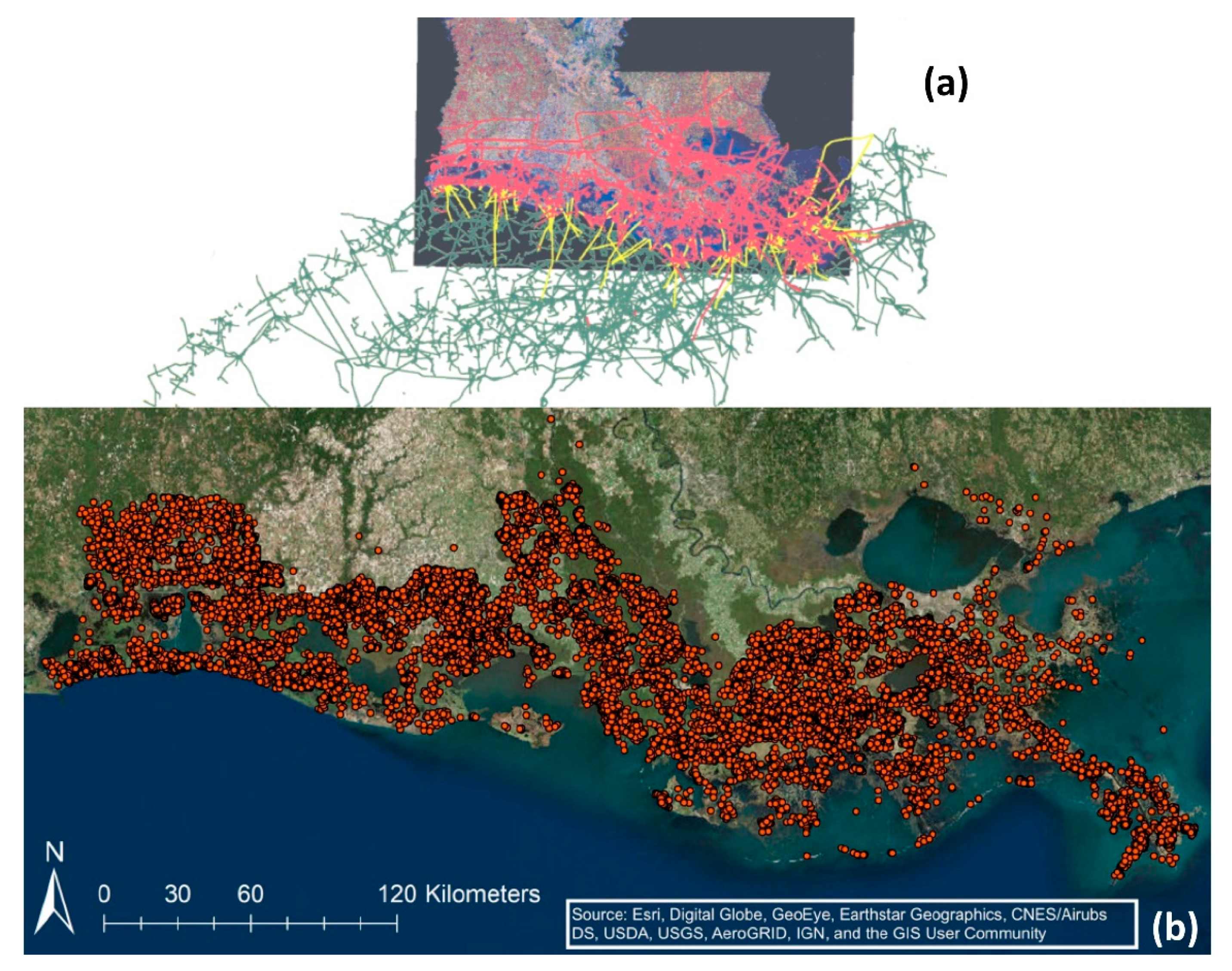The image comprises two distinct, horizontally rectangular sections. The upper section, labeled "(A)" on the top right, features an abstract, colorful depiction set against a dark gray background. This section contains various hues including purples, pinks, blues, and yellows, with numerous blue and green squiggly lines extending downwards.

The lower section, labeled "(B)," is a detailed relief map of the lower half of the United States. This map depicts geographical terrain with varying shades of green and brown, representing land, and blue, representing ocean. The map is marked with numerous red dots all over the coastline, likely indicating data points or availability of a resource. The map also includes a directional arrow pointing north, labeled "N," and a scale ranging from 0 to 120 kilometers. Additionally, there is a white square at the bottom listing sources: ESRI, DigitalGlobe, GOI, EarthStar Geographics, CNES, DS, USDA, USGS, Aerogrid, IGN, and the GIS User Community.